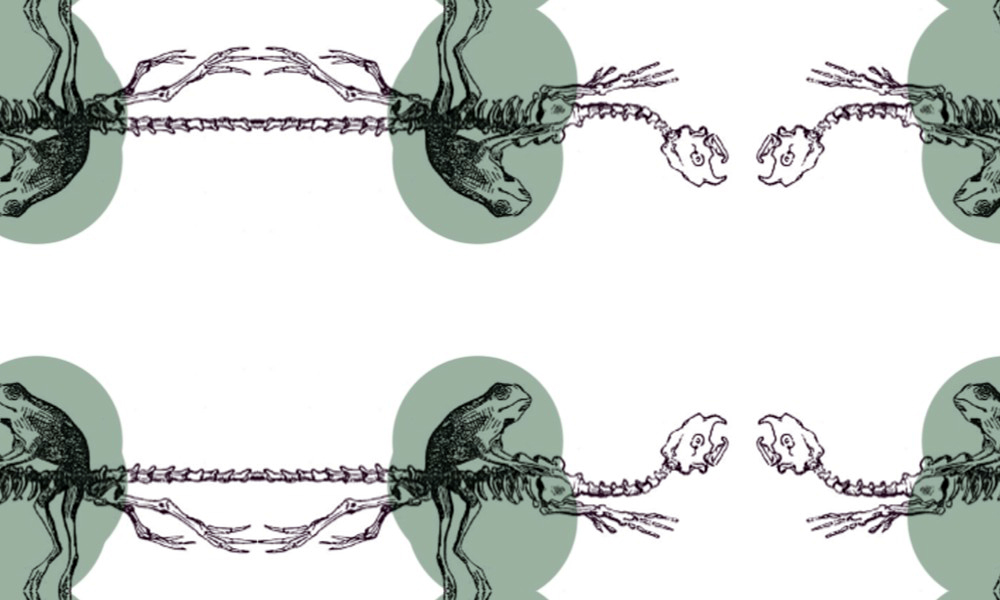The image features a mirrored arrangement against a white background, primarily composed of overlapping green circles, some irregularly shaped. The top and bottom sections of the image reflect each other. Each section includes a black and white depiction of a frog, with the frogs upside down on top and upright at the bottom. 

Prominently, a green circle in the bottom left corner contains a frog depicted mid-jump to the left, while the center circle shows another frog jumping to the right. The bottom right features yet another frog jumping to the left within its green oval. The frogs are interconnected by a prominent, elongated spine, adorned with appendages suggesting legs, hinting at a possible lizard or amphibian structure. A skeleton head and arms are linked to the spine near the center, contributing to the eeriness of the composition. The entire arrangement is digitally crafted, showcasing the frogs, spine, and skeleton in an artfully chaotic yet mirrored pattern, emphasizing a curious blend of natural and skeletal imagery.